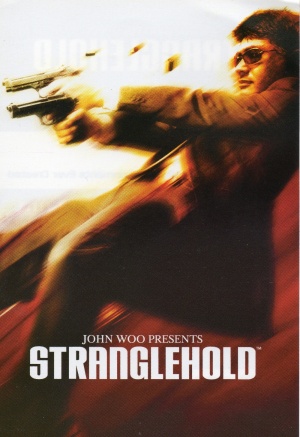This poster, approximately 8 by 10 inches in size, serves as an eye-catching promotional piece for the movie "Stranglehold." The director, John Woo, prominently presents his name in white letters at the bottom, followed by the movie title "STRANGLEHOLD" in bold, uppercase text. 

Dominating the composition is a dynamic profile of an Asian man, possibly of Chinese or Hong Kong descent, whose left side is facing the viewer. He's clad in a long black coat, pants, and sunglasses, with medium-dark hair, embodying an unmistakable image of stylish action. In an acrobatic pose, he is depicted as either leaning or jumping backward while simultaneously wielding two pistols—a black one and a silver or gold one—in a dramatic, cross-armed firing stance. The shell casings are visibly ejecting from the guns, emphasizing the intensity of the scene. 

The background juxtaposes a reddish blur in the lower right and a stark white in the upper left, creating a striking contrast likely enhanced by a yellowish filter over the entire image. A barely discernible watermark consisting of letters spans the top of the poster, adding a subtle layer of complexity to the overall design. This visual spectacle echoes John Woo's renowned style, marked by kinetic action scenes and a flair for the dramatic.